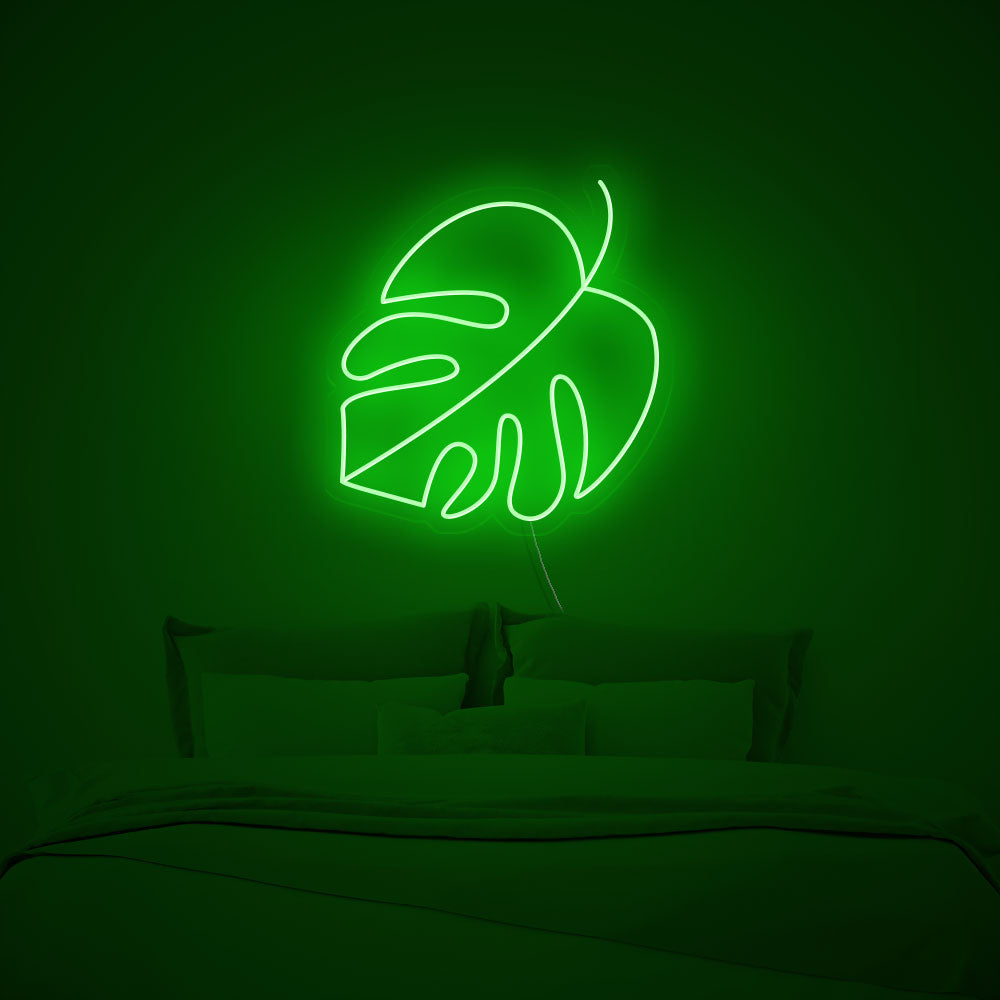This image features a neatly made bed set against a dark room, dominated by the vibrant green glow of a neon leaf-shaped sign mounted on the wall above the headboard. The neon leaf, outlined in bright green light with a stem curving upwards to the right, and detailed with smaller leaves and rounded edges, casts a luminous green hue throughout the room. The bed is adorned with multiple layers of pillows: two large decorative pillows at the back, followed by two white standard pillows, and a smaller, darker decorative pillow in front. The bedspread, either an off-white or tan color, is folded down at the top, exposing the white sheets beneath. A thin white cord from the neon sign is visible, trailing down behind the bed. The minimalist setup emphasizes the glowing neon leaf, making it the focal point of the room, with the green illumination creating a cohesive yet strikingly simple aesthetic.